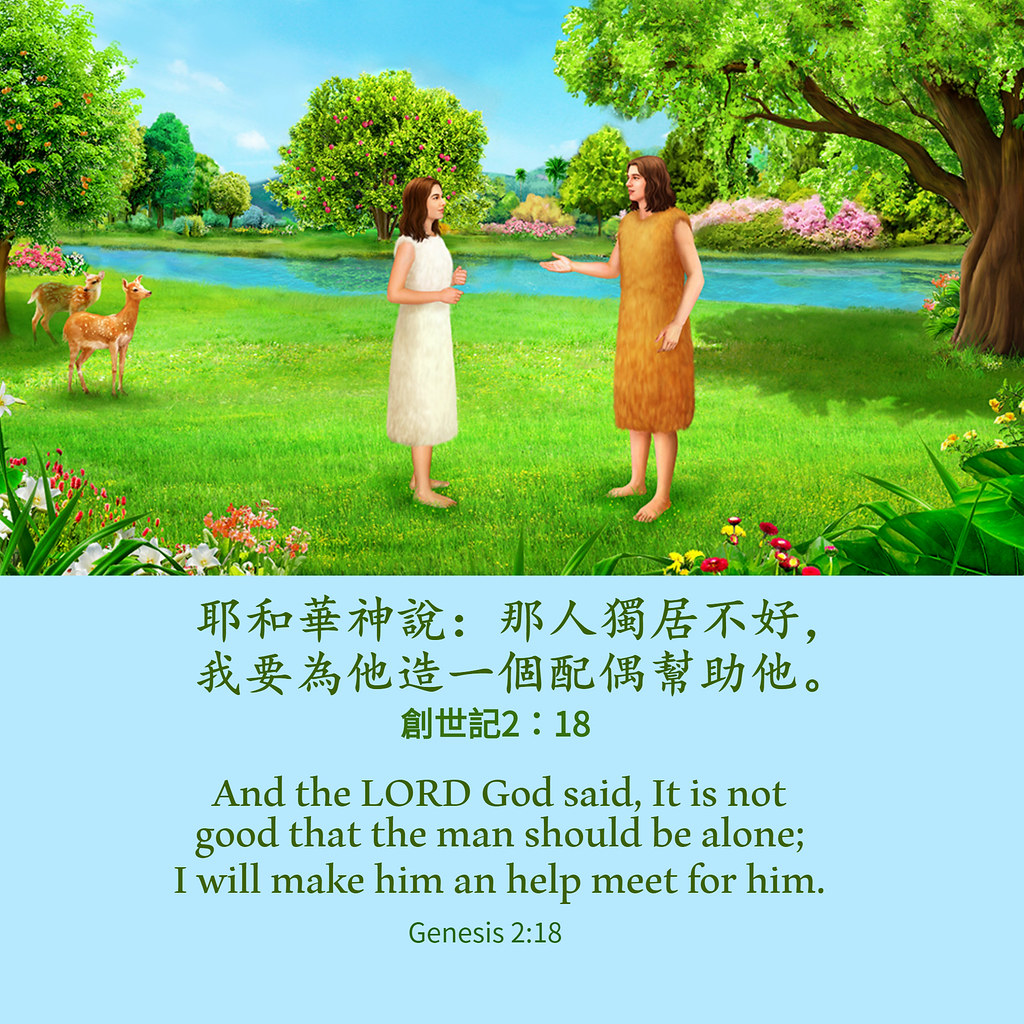The image depicts a vibrant, cartoon-like landscape with two central figures beneath a sky-blue background that features English and Chinese text. In the lush, green environment, an apple tree laden with fruit, an orange tree, colorful flowers, bushes with pink blossoms, and English daisies adorn the scene. A blue stream weaves through a grassy field, adding to the picturesque surroundings. On the left side of the image, two spotted deer fawns graze peacefully.

At the center stand two figures: a woman on the left, wearing a simple white gown, conversing with a taller figure, who might be a man, dressed in a similar brown garment. The backdrop features more trees, possibly with berries or flowers, enhancing the natural beauty of the setting.

The bottom half of the image contains a light blue box with text in both Chinese and English. The English translation reads: "And the Lord God said, 'It is not good that the man should be alone; I will make him a help meet for him.' Genesis 2:18."